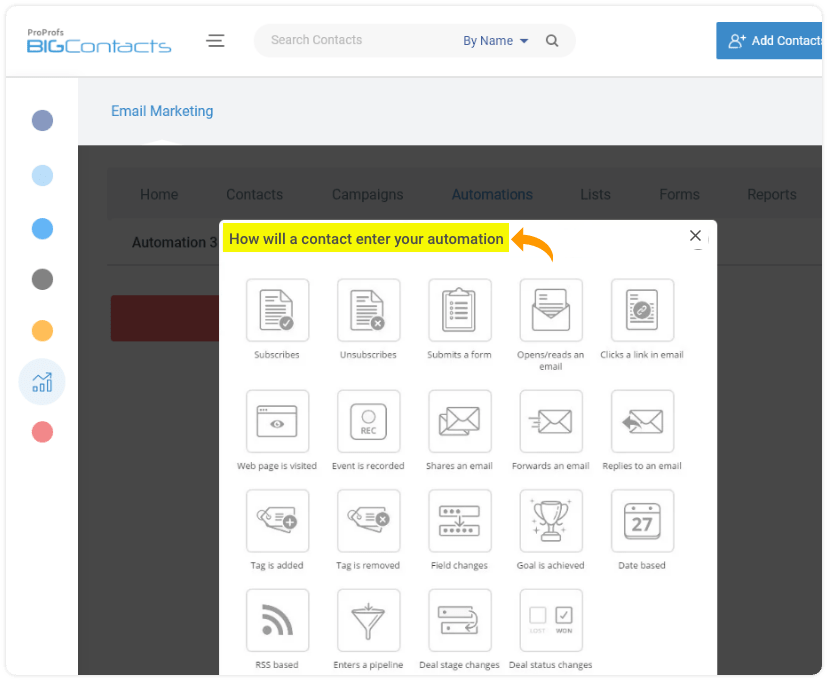The image depicts what appears to be a web interface for ProProfs' BigContacts, a contact management system. In the upper left corner, the words "ProProfs" and "BigContacts" are prominently displayed. "ProProfs" is rendered in a small black font, while "BigContacts" is displayed in a stylized blue font with a computer-like aesthetic.

At the top center of the interface, there is a search bar labeled "Search Contacts." To the right of the search bar is a pull-down menu labeled "by name," accompanied by a magnifying glass icon for initiating searches. Partially visible on the right side of the image is a blue button labeled "Add Contact."

The main area of the webpage is currently grayed out, indicating that a modal dialog box is active. This dialog box contains a header asking, "How will a contact enter your automation?" Below this header, there are multiple tiles, each labeled with different user actions that can trigger automated responses. These actions include "subscribed," "unsubscribed," "submits a form," "opens," "reads an email," and "clicks a link in an email," among other options.

On the left side of the screen, there is a vertical bar featuring colored dots—dark blue, light blue, sky blue, gray, orange, red—and a plus sign above the red dot. These colored dots likely represent different subsets of contacts. Above these dots is a larger circle containing an icon that appears to be a graph, suggesting some analytical or visualization functionality.